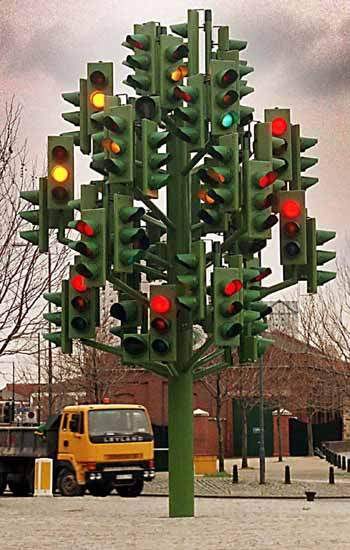The image features a striking sculpture designed to resemble a tree, with a tall green pole serving as the trunk and numerous traffic lights as its branches and leaves. The traffic lights are in varying states, with some showing red, some yellow, and a single green light. This artistic installation is set against a backdrop that includes a yellow Leyland dump truck with a black dumper, positioned near a reddish brick building with a green door panel. Additionally, a yellow and white box is visible in front of the truck. The environment appears to be a busy intersection or square, highlighted by light poles and traffic signals installed on the cobblestone street below. Bare trees devoid of leaves and a gray, overcast sky suggest that the scene is captured in winter.